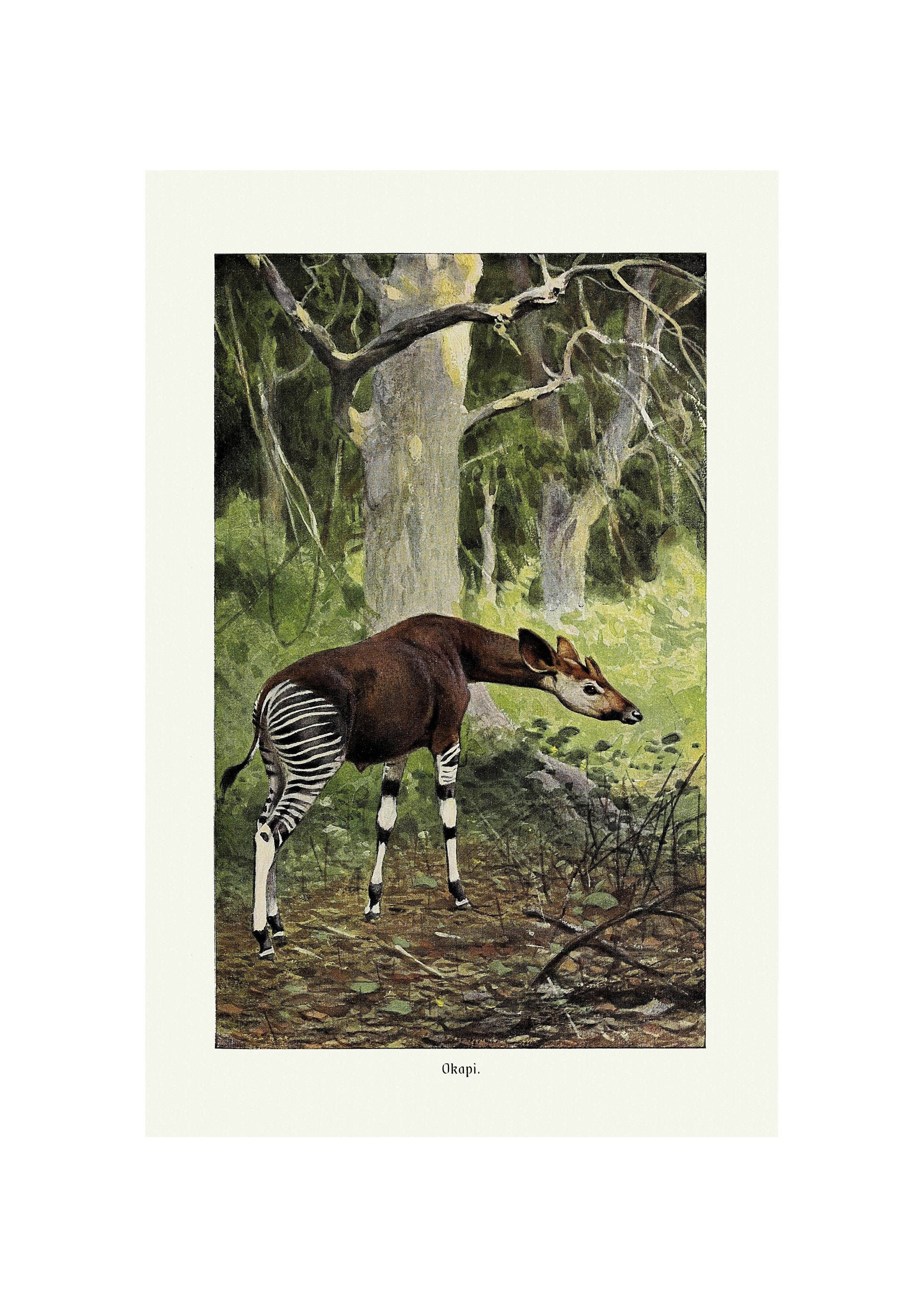This vividly illustrated image showcases a forest scene with a unique, hybrid animal at its center. The animal appears to have the head and upper body of a dark brown deer, complete with large ears and typical facial features. Intriguingly, its front legs, back legs, and rear are striped black and white like those of a zebra. The animal is bent forward, seemingly about to nibble on some tiny, green leaves from low-lying brush and small trees. The surrounding environment is a dense forest filled with vibrant greenery, large oak trees, and patches of brown leaves. The ground is covered with dirt, broken branches, and assorted foliage, with a mix of green grass and other plants dotting the scene. This artistic rendition captures the animal and its woodland habitat in elaborate detail, blending elements of fantasy with natural beauty.